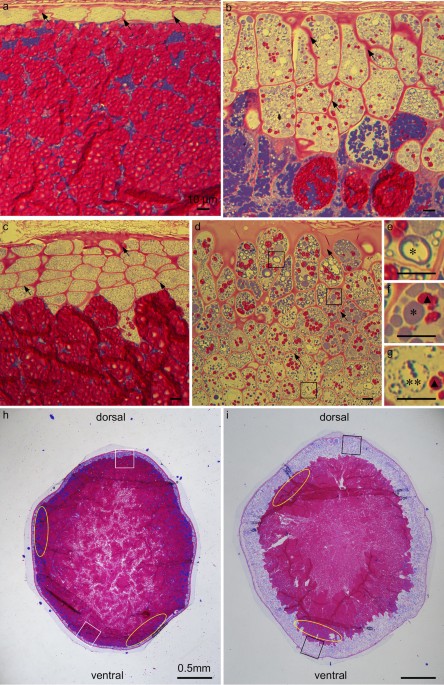This detailed image showcases a collage of microscope slides arranged in a grid, spanning A through I. The slides depict various cellular structures with notable repetition in the pink and tan coloration. Particularly, the bottom two slides, labeled H and I, feature round cells with bright pink central regions, intersected by different colored sections. The left one designates "dorsal" and "ventral" orientations, while the right one is labeled the same. The cells are outlined and segmented, possibly indicating vertebrae or bacterial presence within the muscle tissue.

Further examination reveals diverse morphological details: the slides showcase a range of vivid colors, including prominent reds and yellows, adding to a mosaic-like appearance. Some cells are adorned with blue veins, highlighting internal structures. There's a mix of cell textures, from pixelated and grainy to bumpy patterns, with some cells featuring yellowish fat-like cells interspersed with red dots. The rightmost group of three images, near the bottom labeled dorsal (top) and ventral (bottom), underscores these anatomical orientations.

A significant detail is the presence of measurement markers, specifically one that reads "0.05 millimeters" in black, providing a scale for the microscopic views. Overall, the montage offers an in-depth look at varied cellular and anatomical features through a medical or scientific lens, indicating detailed scrutiny of microscopic organisms or human tissue.